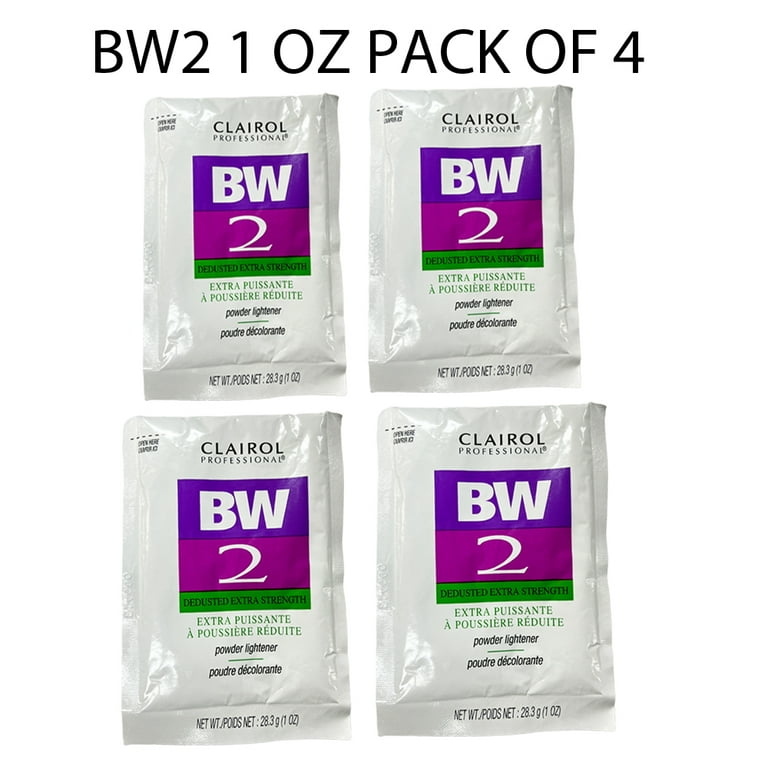The image is a full-color photograph featuring a vertically rectangular layout with no border, set against a white background. At the top, in bold black capital letters, it reads "BW2 1oz pack of 4." Below this title, there are four identical white plastic pouches arranged in a 2 by 2 grid.

Each pouch is labeled with "Clairol Professional" in black font at the top. Centrally, a multi-colored square design is featured; the top band of this square is purple, containing the white letters "BW." Directly below, the number "2" is displayed in white, surrounded by a magenta band. Below this, a thin green rectangle bears the black text "De-Dusted Extra Strength." Furthermore, additional smaller green text reads "Extra Puiciente a Puiciera Rudute," and finally, "Powder Lightener" is printed in black. Additional labeling includes a small green line with "Pudre Decolante" in black font. The total net weight of the contents in each package is 28.3 grams.